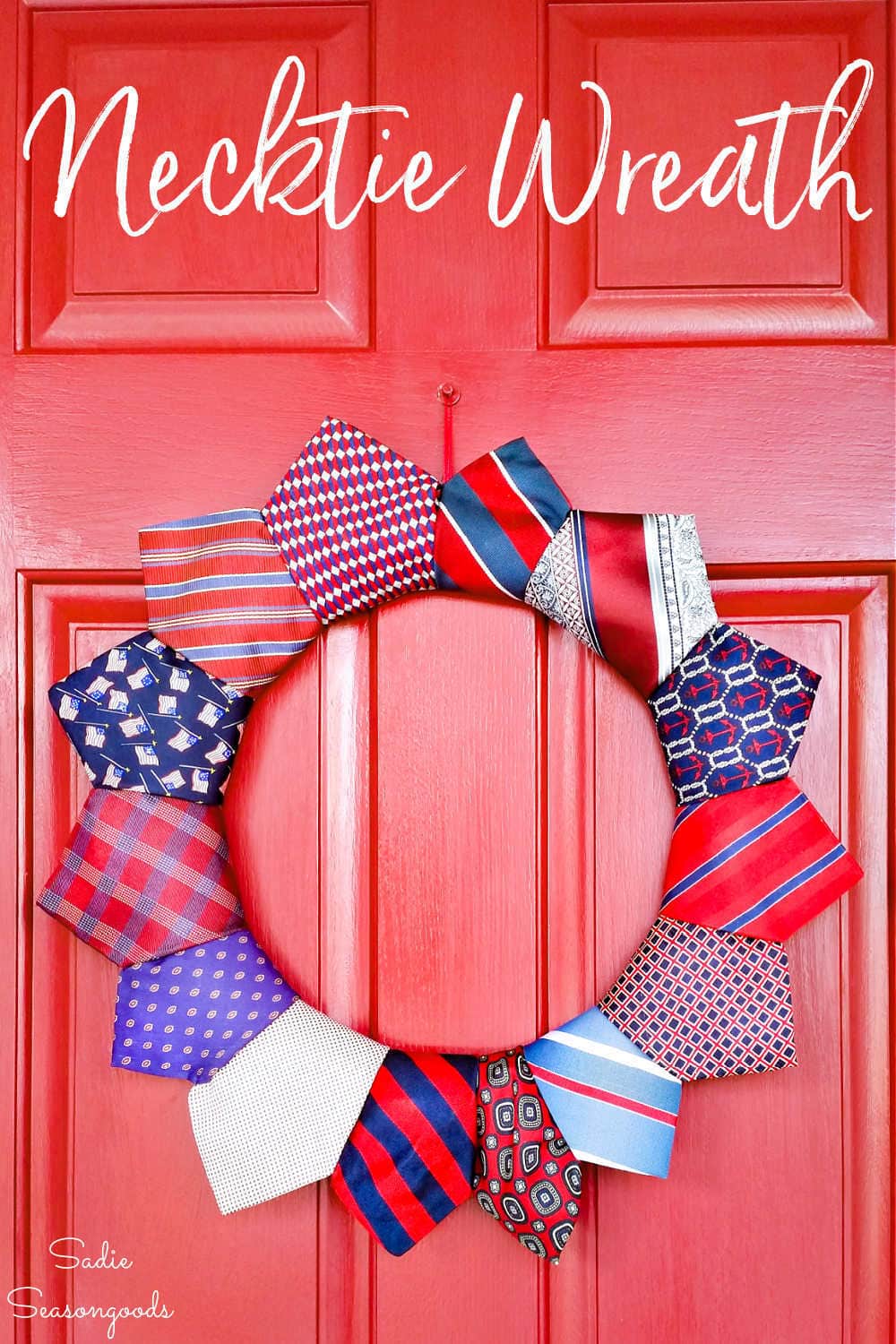The image portrays what appears to be a book or catalog cover with the dimensions of a book cover. Dominating the scene in a portrait orientation is a close-up of a bright red front door. At the top of the door, "Nep-Ti-Reef" is elegantly written in white script-like text, though not all letters are connected. Situated prominently in the center of the door is a creatively designed wreath made entirely from the pointed ends of neckties, each distinct in patterns of red, white, blue, or gray, including plaids, polka dots, and stripes. This unique wreath likely symbolizes the theme "Neck-Tie Wreath," as indicated by the title. In the lower left corner, also in cursive white letters, the name "Sadie Season Goods" is inscribed, suggesting that this cover serves as a catalog for a company that specializes in such creative crafts.